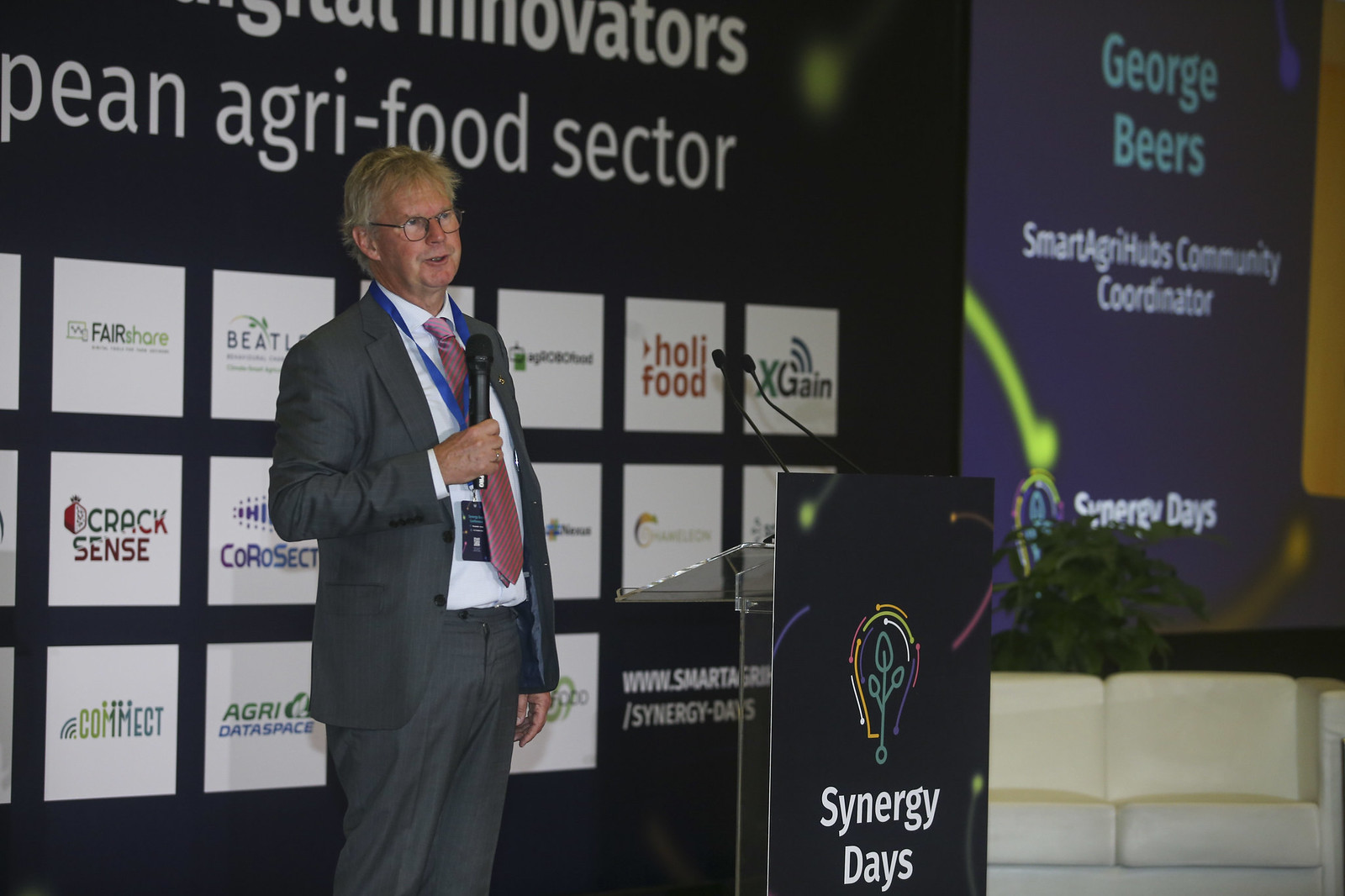The image captures a scene from a seminar, presumably Synergy Days, featuring a man named George Beers, the Smart Agri-Hubs Community Coordinator. He is in his late 60s with disheveled, blondish-gray hair and is dressed in a dark gray suit paired with a pink and gray striped tie. He wears glasses and a blue lanyard, holding a black microphone close to his mouth, indicating that he is in the midst of delivering a speech.

Standing almost close to a podium that is emblazoned with the Synergy Days logo—a light bulb with a plant filament—Beers appears engaged in his presentation. The backdrop is dominated by a black background filled with various logos and inscriptions, including prominently placed signs saying "Innovators P-E-A-N, Agri-Food Sector" and a purple sign identifying Beers with his title. Logos from sponsors like Fair Share, Holifood, X-Gain, Cracksense, Comet, and Agro Data Space are visible, though some text is partly obscured.

Additionally, a white sofa with a green plant behind it is positioned at the far right corner of the stage, adding to the detailed setting of the seminar environment.